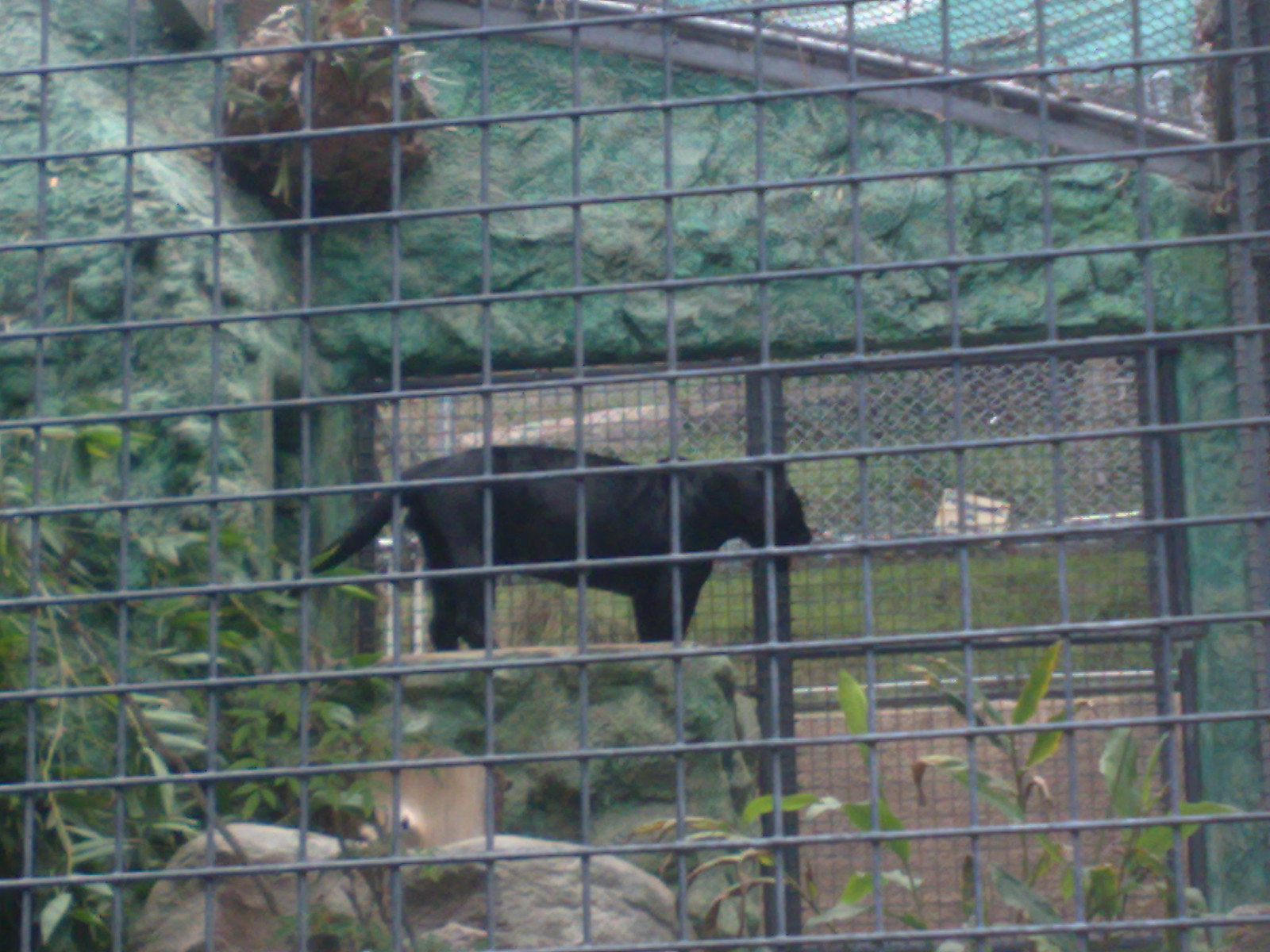This image captures a black panther in a zoo exhibit, seen from the perspective of a visitor standing outside the enclosure. The panther, resembling both a bear and a panther due to its size and demeanor, is positioned prominently, possibly on some rocks, amidst a lush environment with green shrubbery and grassy hills. The enclosure provides ample space for the panther to move around, and it's currently staring intensely, perhaps anticipating feeding time. The background reveals stones, greenery, and a gate further in the distance, suggesting the exhibit is quite expansive and not located in the United States. This photograph conveys the panther's powerful presence and the zoo's effort to mimic its natural habitat within captivity.